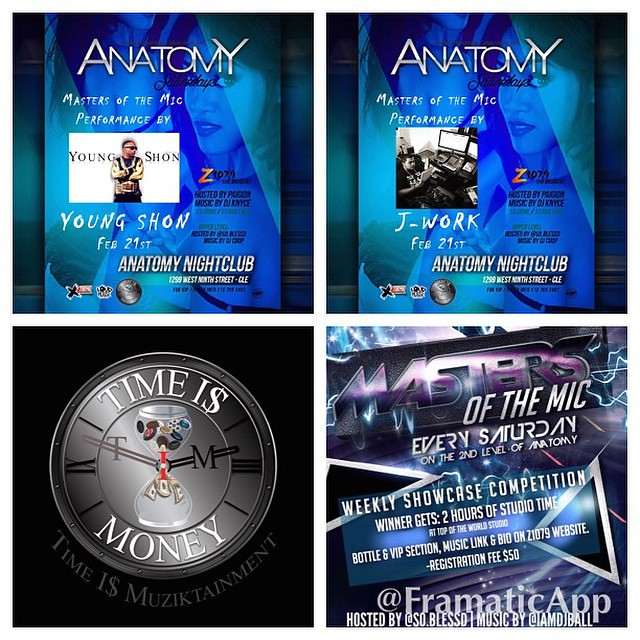This square image showcases four distinct square posters arranged in a 2x2 grid, separated by thick white lines. The top two posters are identical, featuring a blue and green background adorned with images of women, overlaid with silver and white text. At the top of these posters, in silver font, the word "Anatomy" is prominently displayed, followed by the event title in white font: "Masters of the Mic." Beneath this, the posters announce a performance by "Young Sean" scheduled for February 21st, accompanied by a white silhouette of a rapper. 

The bottom left poster features a black background with a gray clock image showing a time between 2:00 and 2:30 and adorned with the phrase "Time is Money" in white letters, where the 'S' is stylized as a dollar sign. Around the clock face, it reads "Time is Musictainment."

The bottom right poster has a gray-blue background with silver accents and contains the phrase "Masters of the Mic" in white letters. It details a weekly showcase competition held every Saturday on the second level of a venue, annotated with "@FormaticApp" and additional hosting details. 

Overall, each poster stands out with unique colors and designs, promoting different themes centered around music and performance.